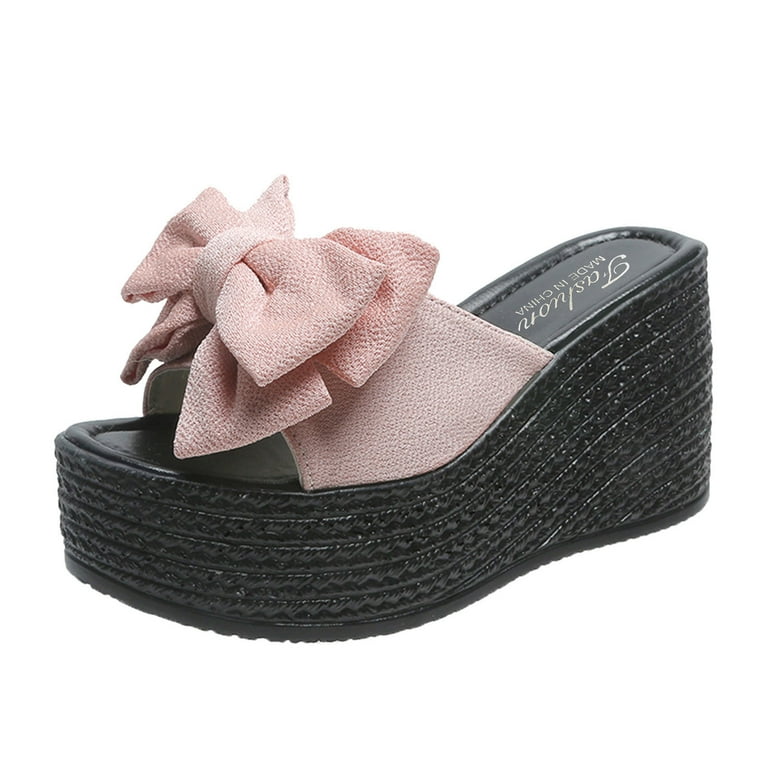This close-up image features a single left high-heeled platform wedge sandal, prominently displayed against a stark white background. The shoe's thick, solid wedge base, approximately four inches tall, is predominantly black with ridged detailing along the sides of the sole, providing a sturdy foundation. A delicate, light pink band, which transitions into a large, ostentatious bow at the top, adorns the sandal. This bow is flanked by two additional ribbon-like extensions, creating the effect of a triple bow design. Inside the sandal, the black sole features the brand name "Fasluan" and a "Made in China" label, both inscribed in white or tan lettering. The stitching on the sandal is black, and there's a shiny white accent along the side, contributing to its stylish aesthetic. This intricate combination of black and pink elements gives the shoe a striking and fashionable appearance.